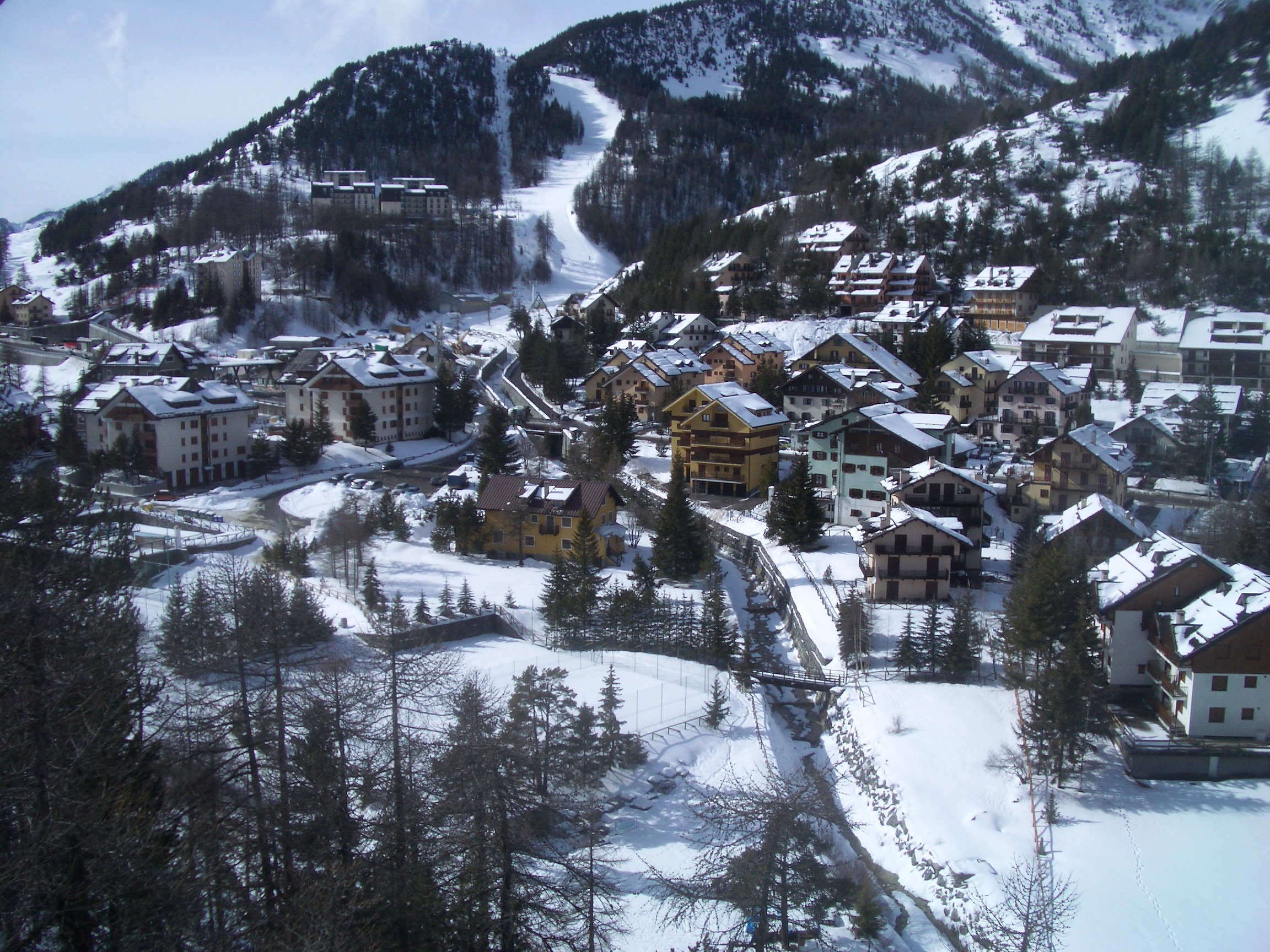A stunning winter scene captures a picturesque ski town nestled at the base of a snow-covered mountain. The town's architecture is a charming blend of tall houses and apartment buildings, with some homes perched halfway up the mountain. These buildings are arranged at various angles, adding to the town's quaint and cozy atmosphere. The freshly fallen snow blankets the entire landscape, lending a crisp, clean look to the scene.

A ski slope carves its way down the mountain, paralleled by what appears to be a chairlift track, making this a popular destination for winter sports enthusiasts. The mountain’s inclines and the valley nestled between peaks are strikingly beautiful under the clear, sunny sky. Sunlight glistens off the snow-covered rooftops and trees, which vary in size and add depth to the landscape.

A road winds through the town, disappearing underneath a pedestrian overpass and eventually leading towards what is likely a ski resort. Near the condo area, a small parking lot holds a few parked cars, suggesting visitors have already hit the slopes. The overall scene is tranquil and inviting, capturing the essence of a perfect winter getaway.